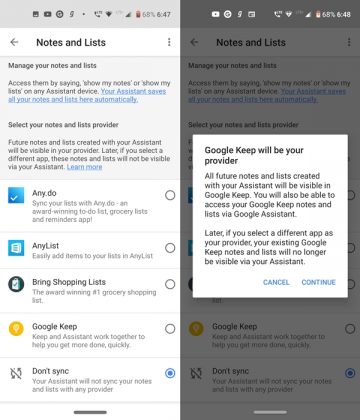**Caption: Detailed Comparison of Two Application Screenshots Featuring Note and List Management Options**

The image showcases two side-by-side screenshots of a note and list management application. 

- **Left Screenshot:**
  - **Background:** Predominantly white with a thin gray border.
  - **Top Bar:** Displays standard time, battery, and Wi-Fi icons in black.
  - **Header:** Features a black arrow pointing left, labeled "Notes" in bold black font, with "Lists" on the right. To the far right, there is a vertical ellipsis (three vertically aligned black dots).
  - **Blue Section:** Occupies the top portion with the heading "Manage notes and lists" in bold black text. Below, it instructs the user to select a notes and list provider with additional information provided.
  - **Content:**
    - Listed providers with matching icons on the left and right:
      - **Any.do:** Icon on the left, followed by its name in black and three lines of information.
      - **AnyList:** Similar format with one line of information.
      - **Bring Shopping Lists:** Icon on the left, its name in black, and two lines of information.
      - **Google Keep:** Same format, two lines of information.
    - The icons are encased in white circles with gray borders, except for the last one, which is blue.

- **Right Screenshot:**
  - **Background:** Grayish due to a pop-up overlay.
  - **Content:** Identical to the left screenshot except for the addition of the pop-up.
  - **Pop-Up:**
    - **Top Left Corner:** Bold text stating "Google Keep will be your provider."
    - **Body:** Two paragraphs of information explaining the selection.
    - **Bottom Right Corner:** Features a "Continue" button in blue, with a "Cancel" option in blue to its left.

Both screenshots offer a comparative view of the interface with and without the selection pop-up, providing a comprehensive illustration of the application’s note and list management options.